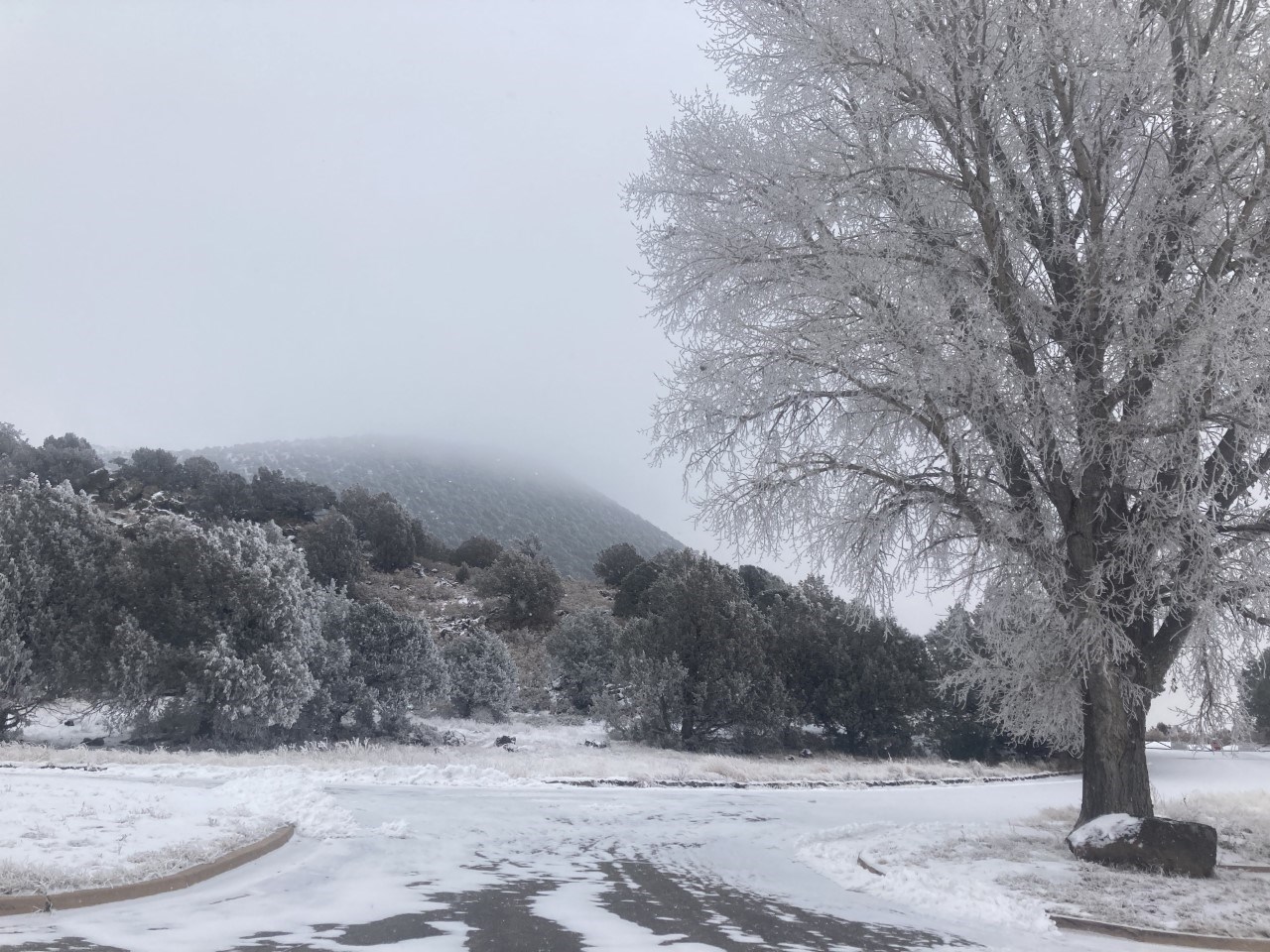The photograph captures a serene winter scene, taken from the center of a snow-covered road. White snow blankets the black pavement, with patches of grass peeking out near the curbs. Dominating the right hand side is a large tree, stripped of leaves and adorned with frozen branches. The background features a dense, snowy woodland area extending up a heavily wooded mountain, whose peak is shrouded in fog that merges seamlessly into the overcast, gray sky. Despite hints of green from scattered evergreen trees, the pervasive snow lends the image a nearly black-and-white appearance, enhancing the overall dreary, grayscale ambiance.